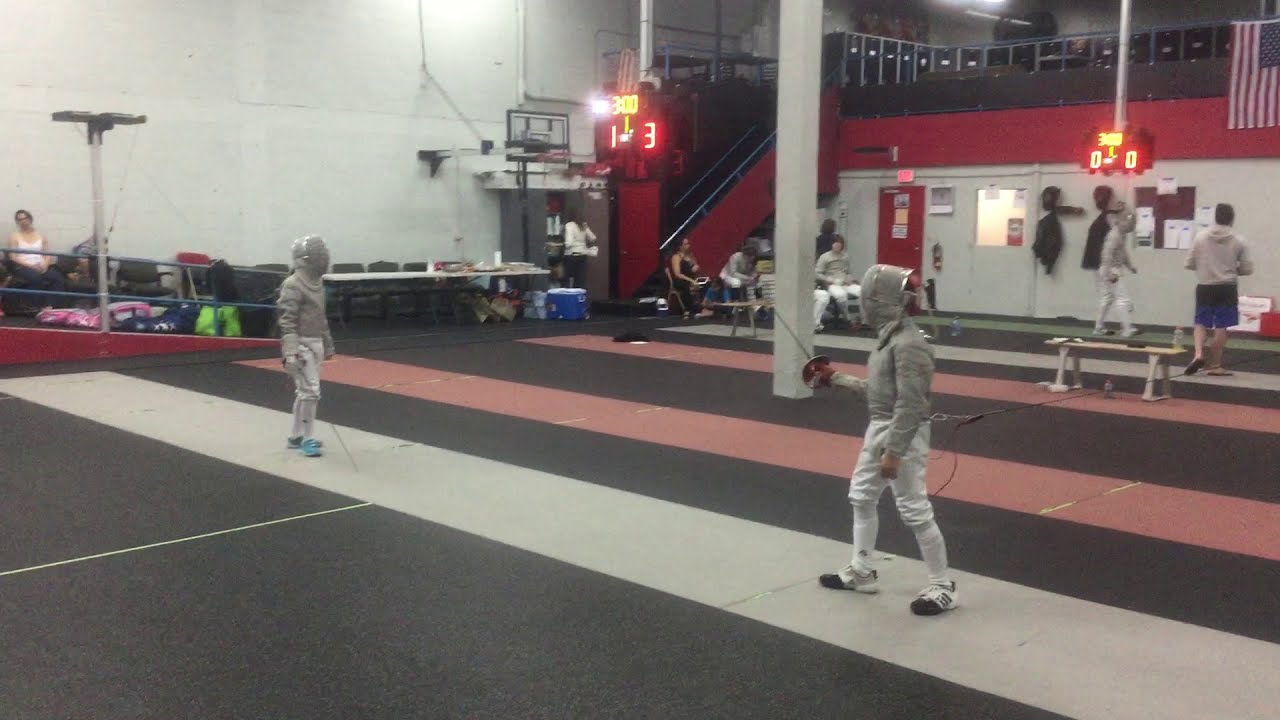This horizontally aligned rectangular picture captures an indoor fencing gym, featuring two fencers in action. The spacious gym, characterized by its white walls and a white column in the middle, also has black and red painted sections adding contrast. At the upper right corner, a digital scoreboard displays zero for both sides, illuminated with a time of 3:00. The floor is padded, consisting of variously colored stripes in no particular pattern, including gray, white, pink, red, and a mix of other colors.

The two fencers, positioned almost symmetrically at the center of the image, face each other with swords in hand, dressed in typical fencing attire: gray long-sleeved tops, white pants, and gray masks. Behind them, a woman in a white tank top sits against the white wall amongst chairs lined up behind a table. The scene also includes a stairwell to the left, with various other spectators and objects subtly populating the background, adding to the overall depth and detail of the setting.